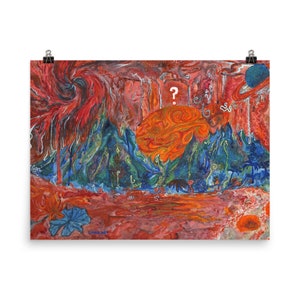This is a small, square image of an abstract painting, highlighted against a larger white background and secured with black binder clips in the top left and right corners. The painting features bold, exaggerated brushstrokes with swirls of red, orange, and blue dominating the piece. At the center of the image, jagged mountain peaks in shades of blue and green rise up, forming a valley-like depression. Above these peaks, an orange circular object with red swirls—the sun—occupies the middle of the painting. Notably, a white question mark has been painted on this sun. The landscape beneath the mountains is filled with vibrant red and orange hues, while the sky above continues the theme with swirling red, orange, and blue lines, creating a dynamic and evocative scene without any discernable signatures.